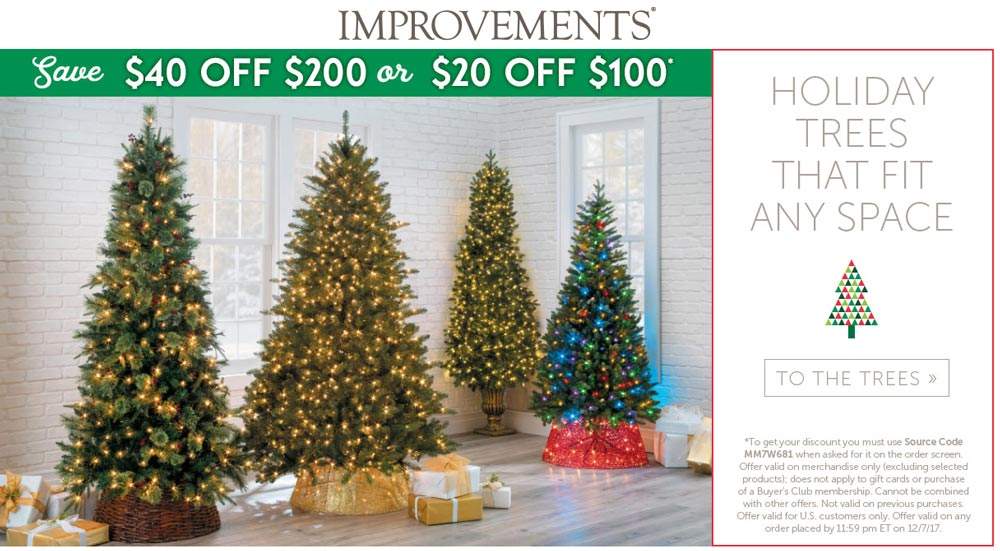The image displays a website called "Improvements," with the name prominently written in a sleek grey font across the center. Below the title, a vibrant green banner advertises promotional offers: $40 off purchases of $200 or more, and $20 off purchases of $100 or more. Beneath the banner, there is a cozy indoor scene featuring four illuminated Christmas trees of various styles, each standing in a festive arrangement with a scattering of wrapped presents at their bases.

To the right of this main image, within a box outlined by a thin red line, large, capitalized text reads: "HOLIDAY TREES THAT FIT ANY SPACE." Adjacent to this text is an image of a one-dimensional Christmas tree adorned with lights. Below this visual, there is a clickable button or link for visitors to explore more detailed information about the available Christmas tree options.

At the bottom of the page, a paragraph of explanatory text details the conditions for the promotional discounts, instructing customers on the necessary steps to redeem the offered savings.